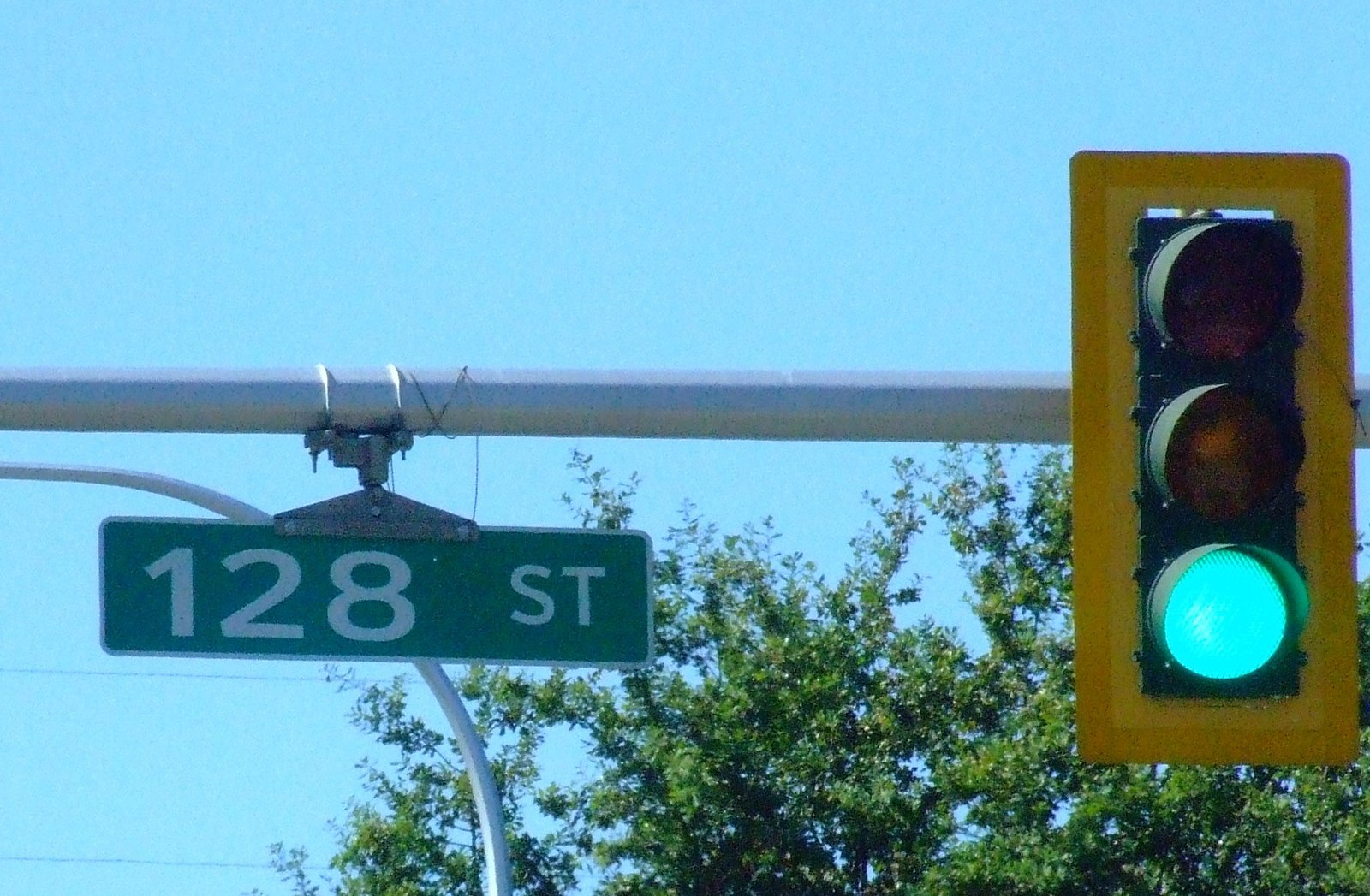This photograph vividly captures a vibrant street scene under a clear, deep blue sky. Dominating the image is a silver pole, positioned slightly off-center, which supports a green street sign that reads "128th Street" in bold white font. This sign is fixed to the pole with a visible pipe clamp. Just above and extending towards the right, an arched light pole comes into view. In the far right of the image, a typical traffic light is suspended, its bright yellow frame encasing the standard red, yellow, and green lights, with the green light illuminated. Below and stretching towards the bottom right corner, a lush, fully leafed out green deciduous tree fills the remaining space, providing a vibrant contrast against the sky. The overall composition and brightness suggest it is a sunny summer day, free from clouds.